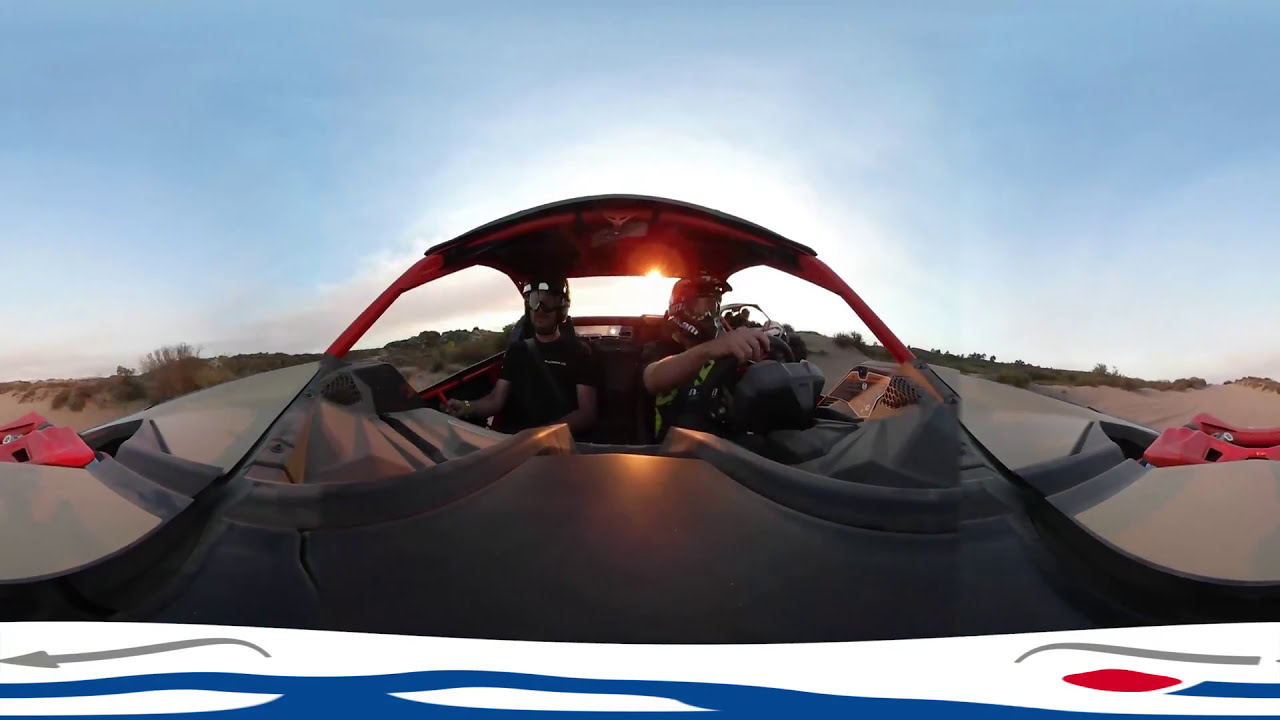The image features a 360-degree view taken from the front hood of a dune buggy driving through a sandy desert terrain. The vehicle has an oddly shaped design, with a black hood and a red metal roof frame. The dune buggy is open-sided with no windows, allowing a clear view of the desert landscape which includes sand, wispy grass, and some patches of vegetation. The driver, positioned on the right, is wearing a full head helmet with a mask and goggles, while the passenger on the left is donning a black t-shirt, a partial helmet, and goggles. Both individuals are holding onto the buggy, indicating the motion of their ride. The sun is visible through the back of the vehicle, casting a warm glow over the scene, with a blue sky and scattered white clouds overhead. Additionally, a small part of another buggy is visible just to the right of the main vehicle. The image includes a white banner with some gray, blue, and red shapes at the bottom, adding to the dynamic nature of the composition.